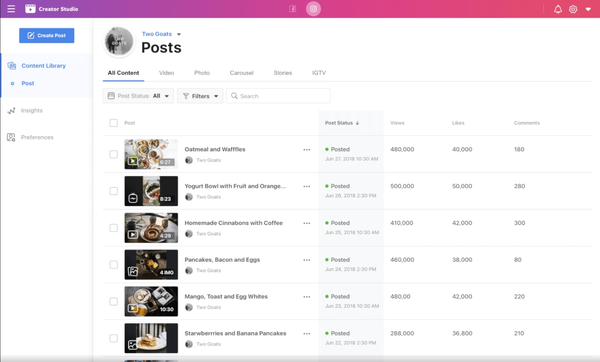Here is a detailed and cleaned-up descriptive caption for the image:

"This screenshot captures the interface of Creator Studio for Facebook and Instagram. Dominating the top of the page is a gradient banner that transitions from purple on the left to reddish on the right. The banner is labeled 'Creator Studio' on the left side and displays both Facebook and Instagram icons in the center. On the right side of the banner, there is a bell icon, a widget symbol, and a downward-facing arrow.

Running vertically down the left side of the page is a panel with various options, including ‘Create Post,’ ‘Content Library,’ ‘Posts,’ ‘Insights,’ and ‘Preferences.’ On the right side of the page, there is a list of videos. At the top of the list are a round profile picture and the text 'Two Goats,' accompanied by a downward-facing arrow next to 'Posts.'

Below this, there is a navigation bar with options for different types of content: ‘All Content,’ ‘Video,’ ‘Photo,’ ‘Carousel,’ ‘Stories,’ and ‘IGTV.’ Beneath this navigation bar, six lines detail recent video posts. Each line lists one video, accompanied by a thumbnail photo on the left depicting the food in the video. The videos and their corresponding details are as follows:

1. 'Oatmeal and Waffles,' posted on July 27, 2018, at 10:30 AM
2. 'Yogurt Bowl with Fruit and Orange,' posted on July 26, 2018, at 2:30 PM
3. 'Homemade Cinnabons with Coffee,' posted on June 25, 2018, at 10:30 AM
4. 'Pancakes, Bacon and Eggs,' posted on June 24, 2018, at 2:30 PM
5. 'Mango Toast and Egg Whites,' posted on June 23, 2018, at 10:30 AM
6. 'Strawberries and Banana Pancakes,' posted on June 22, 2018, at 2:30 PM

Each video's thumbnail prominently displays the culinary delights mentioned, capturing the essence of the post."